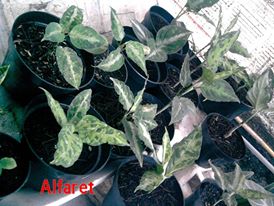The image features several small houseplants, with at least five or six black plastic pots, rather than the previously mentioned green pots. These pots are placed close together on a windowsill, which is illuminated by natural sunlight streaming through white blinds. The plants predominantly display green leaves marked by distinct white stripes, and some leaves exhibit dot-like patterns. In the bottom left corner of the picture, the word "alpharet" is prominently written in red. The varying shapes of the leaves include both oval and triangular forms, complementing the overall lush, verdant scene. The backdrop of bright daylight enhances the greenery, highlighting the thriving nature of these non-flowering plants.